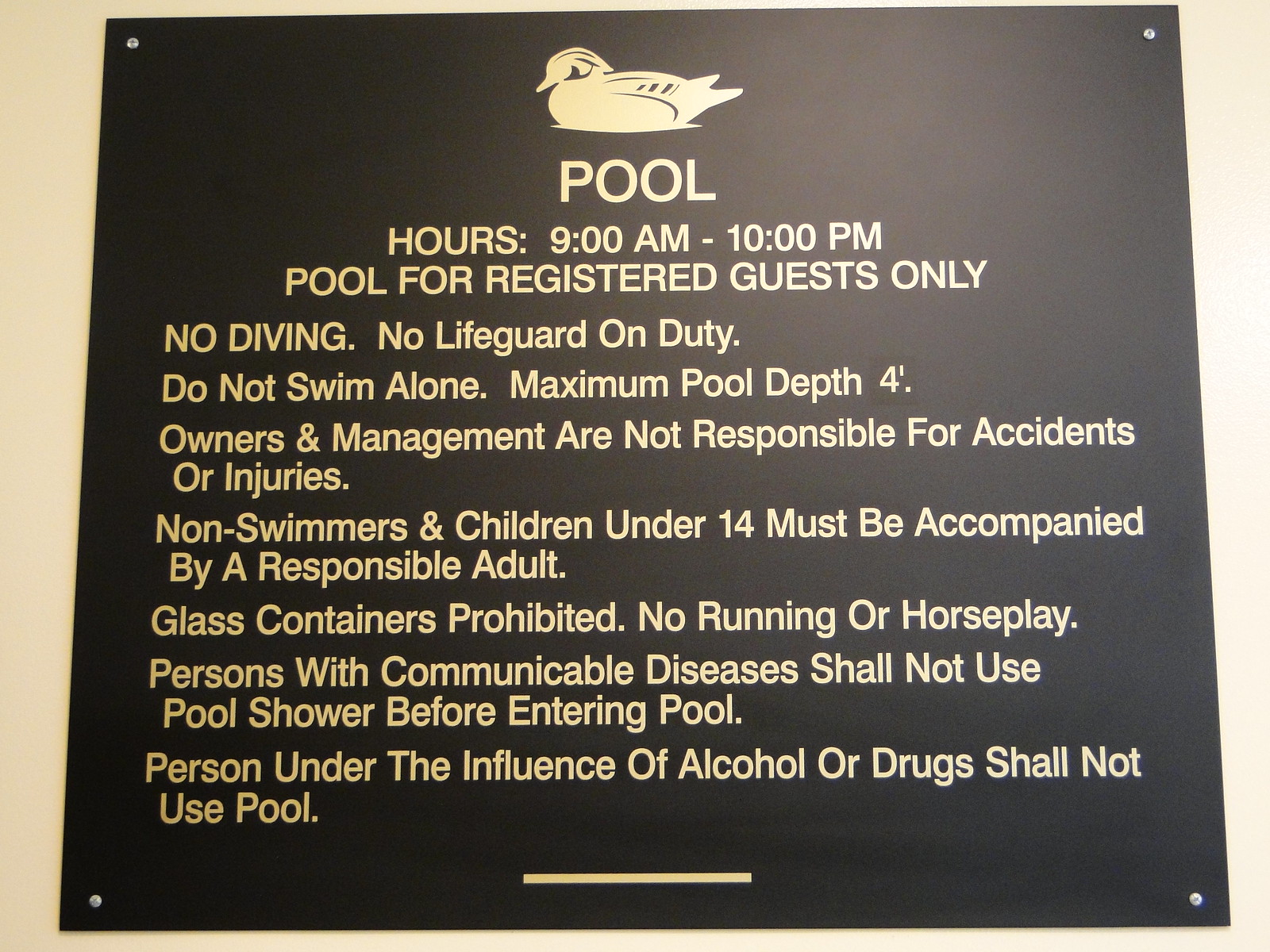This detailed photograph displays a square-shaped plaque mounted on a light-colored wall, affixed with screws in its corners. The plaque is prominently brown with yellow or gold inscriptions. Dominating the top section is an image of a bird, possibly a duck or swan, facing left. Directly beneath this, in bold, large capital letters, the word "POOL" is inscribed. Below this, several informative lines follow, providing essential regulations and instructions:

- "Pool Hours: 9 am to 10 pm"
- "Pool for Registered Guests Only"
- "No Diving"
- "No Lifeguard on Duty"
- "Do Not Swim Alone"
- "Maximum Pool Depth: 4 Feet"
- "Owners and Management Are Not Responsible for Accidents or Injuries"
- "Non-swimmers and Children Under 14 Must Be Accompanied by a Responsible Adult"
- "Glass Containers Prohibited"
- "No Running or Horseplay"
- "Persons with Communicable Diseases Shall Not Use Pool"
- "Shower Before Entering Pool"
- "Persons Under the Influence of Alcohol or Drugs Shall Not Use Pool"

The text at the bottom of the plaque is capped off with a short, horizontal line centered at the very bottom. The sign’s legibility and the presence of indoor lighting suggest it is mounted inside, perhaps in a hotel's basement or roof area.